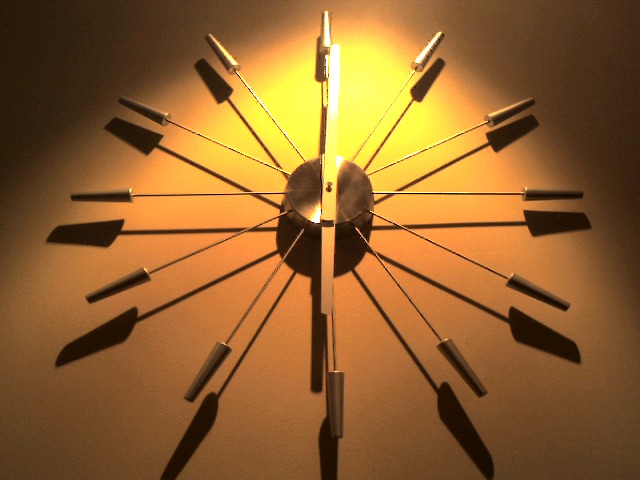The image portrays a highly modern and futuristic wall clock mounted on a gradient backdrop that transitions from a dark yellow at the bottom to a brighter yellow in the upper area, accented by an orange semicircular line. The clock is distinctly unconventional, featuring no letters or numbers. It consists of multiple slender metal rods radiating outward from a central gold disc, each rod ending in a thicker, brownish tip. These rods seemingly represent the positions of traditionally numbered hour markers. The clock's hands are simple yet elegant gold metal pieces, with one aligned vertically to mark the hour and minute. Additionally, there is a visible shadow cast by the clock’s hands, adding depth to the image. The overall design exudes a sophisticated, avant-garde aesthetic.